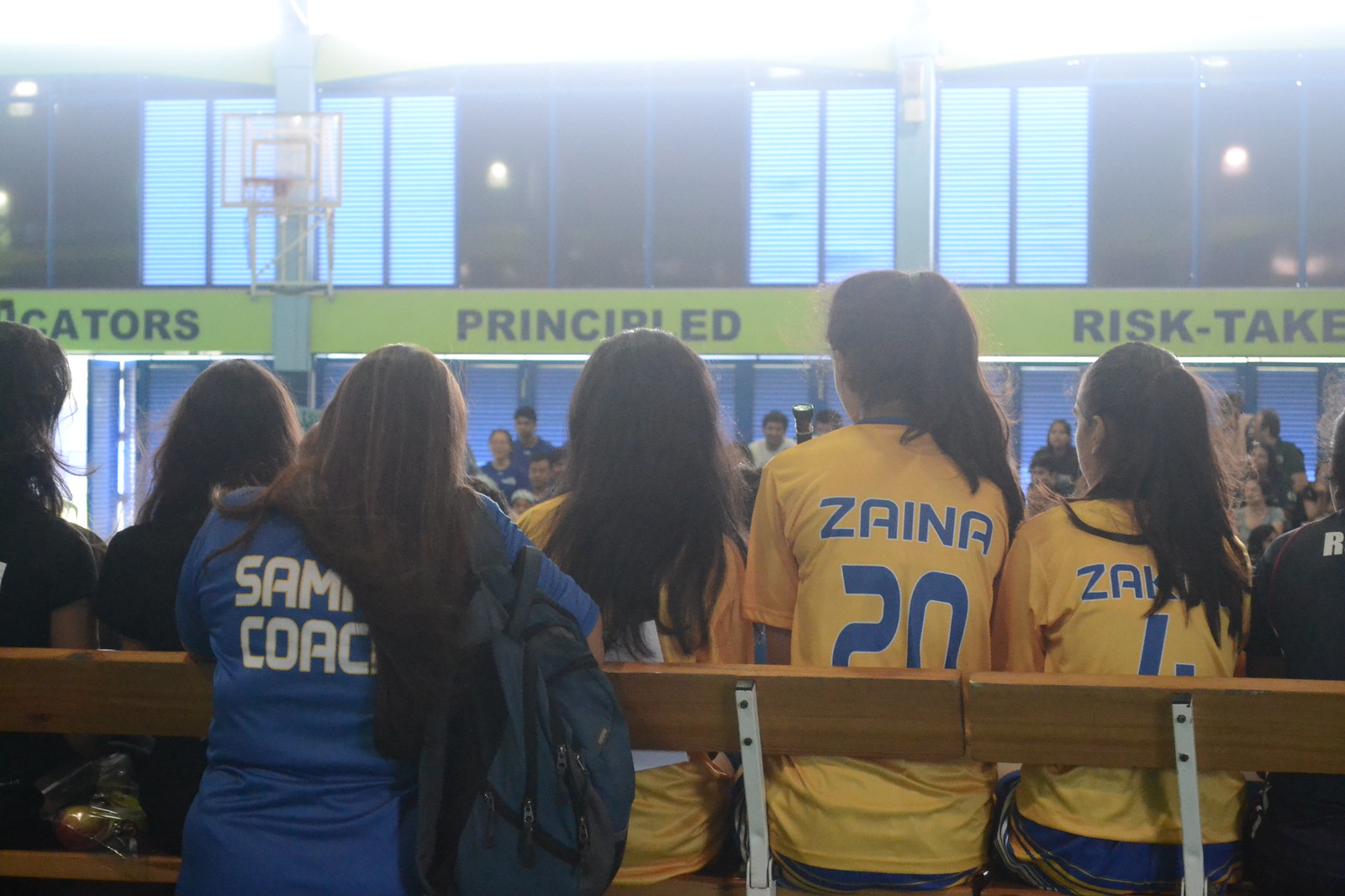In a bustling gymnasium, a group of young girls, all sporting long black hair, sit together on a bench, intently watching a basketball game. Most of the girls are dressed in yellow jerseys with the name "Z-A-I-N-A" emblazoned on the back, each accompanied by unique blue numbers. One noticeable girl in the middle wears a blue shirt instead, with her name partly obscured by her long hair. To her left, a woman stands, donning a blue shirt with the partial name "S-A-M" visible, followed by the word "Coach" in white letters. She carries a backpack over her right shoulder. A sign in front of them reads "Gators: Principled Risk Takers" in green with blue lettering, surrounded by a large crowd of spectators also engrossed in the match. The gym is highlighted by a basketball hoop on the left side, positioned in front of a window, while another window is visible on the right. Above the top level of the gym, black letters spell out an indiscernible message, reinforcing the energetic and organized atmosphere of the space.